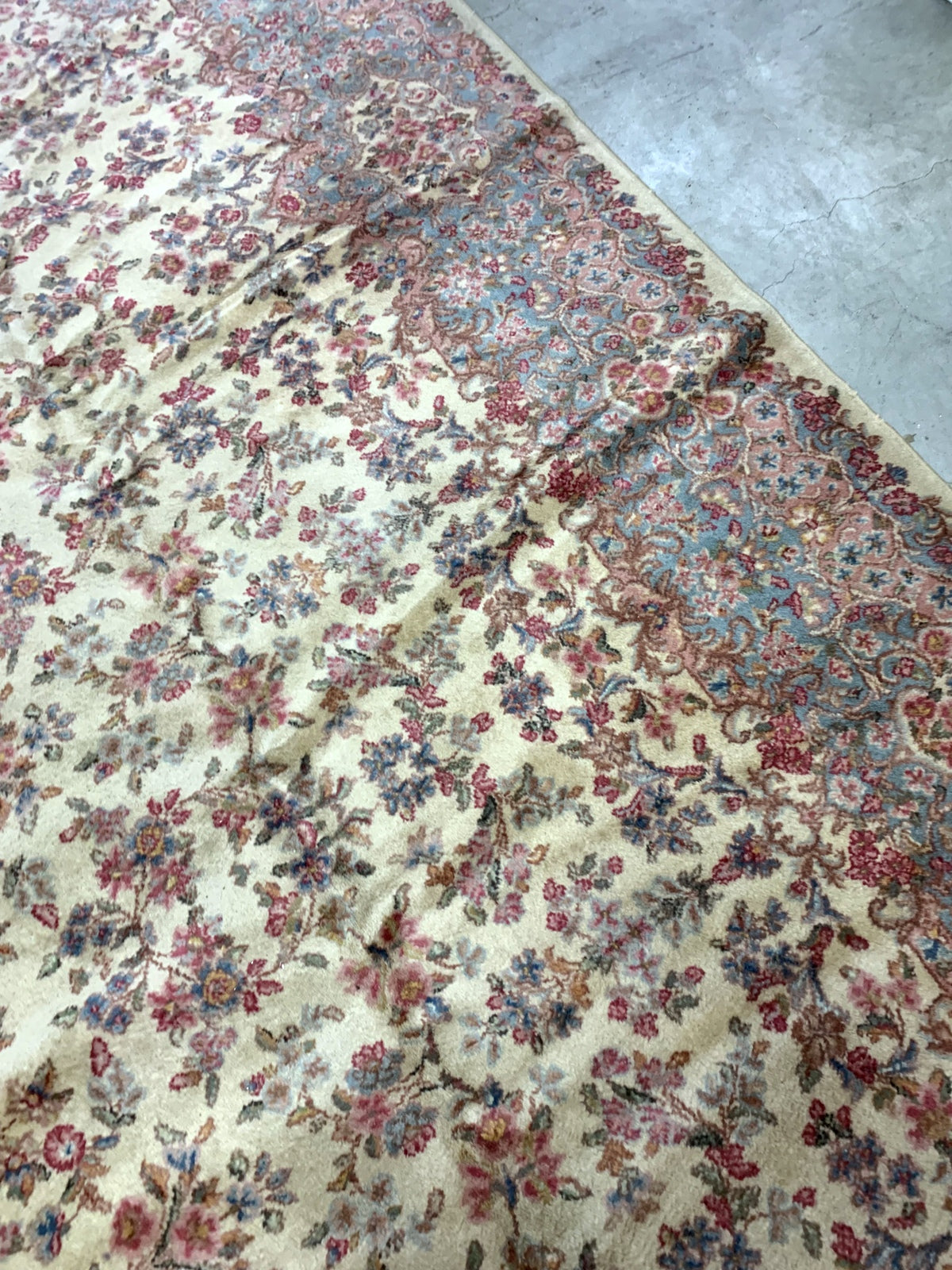This portrait-oriented close-up photograph captures a richly detailed, floral area rug laid diagonally across a bare gray stone floor. The rug is predominantly cream-colored with a luxurious golden beige hue. The intricate floral pattern features an array of colors, including deep reds, pinks, blues, light purples, and shades of green, with elements of burgundy and gray. The flowers, resembling roses and other types, densely decorate a thick outer border while becoming sparser towards the center. The rug's left and bottom edges extend out of the frame, while the top right corner highlights a noticeable triangle of the gray floor, giving a sense of its unique placement.